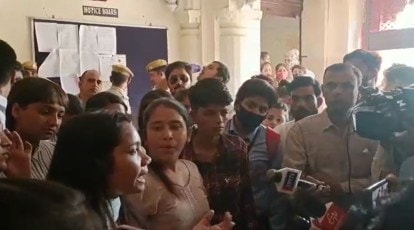In the image, a large group of about 20 people, predominantly of Indian descent, are crowded into a cream-colored room with a chalkboard and various sheets of paper pinned to a bulletin board on the left side. Above the chalkboard, there is an inscription in a foreign language. In the background, light pours in through a window located in the upper right corner, and a few individuals, including men in uniforms with tan berets, are seen standing near a doorway. 

In the foreground, a woman with dark hair appears upset, possibly yelling or speaking loudly, while several people hold microphones towards her and a large video camera is pointed at her. The focus of the room is clearly on this woman, as most individuals are looking and listening attentively to her. Some people in the image, including a person wearing a black mask in the center, add to the sense of tension and urgency in the scene.